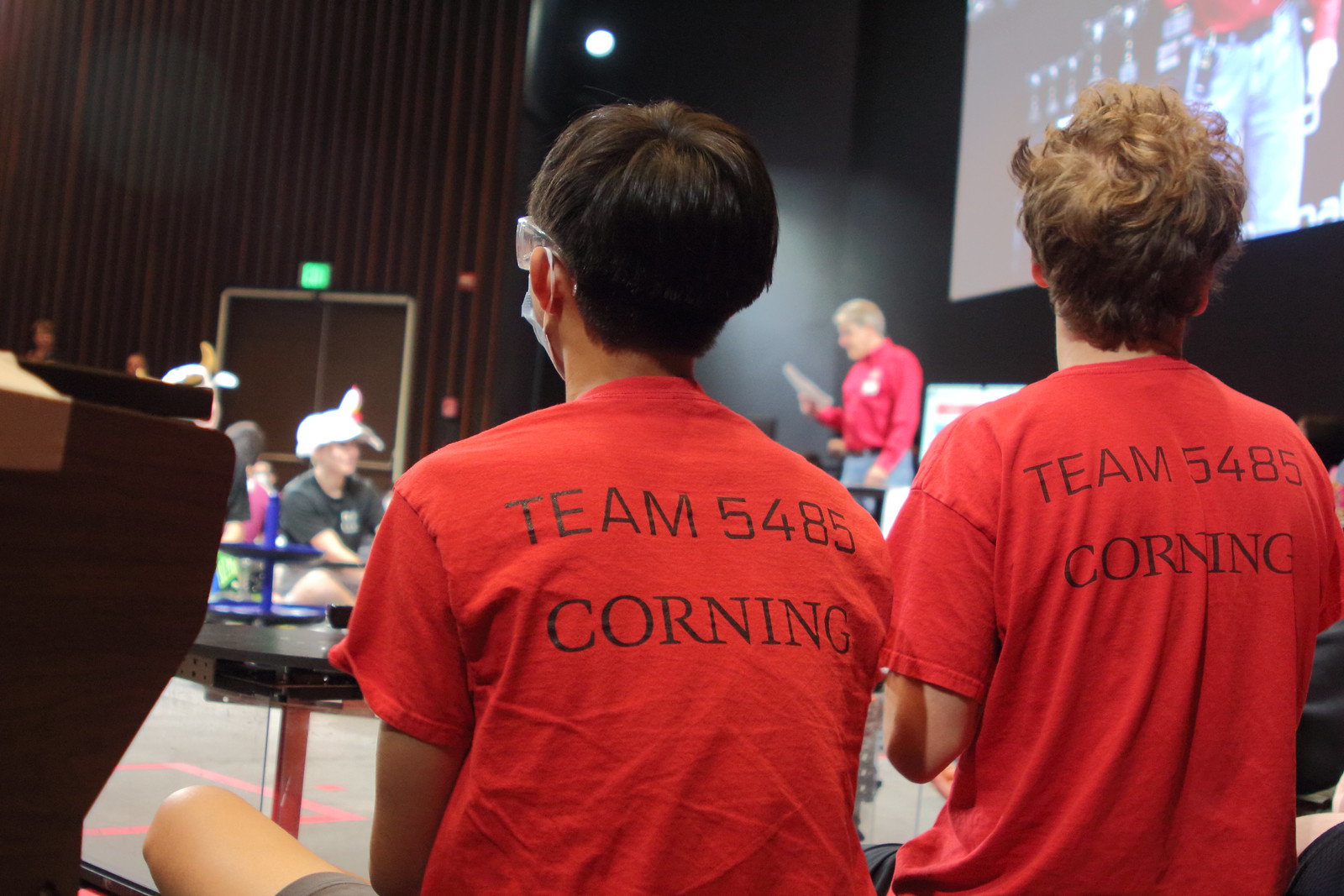In this color photograph, we see the backs of two individuals, possibly young males, seated in what appears to be an auditorium during a contest or tournament. Both are wearing bright red shirts labeled "Team 5485 Corning" in black text. The person on the left has short, dark brown hair and is also wearing protective glasses and a COVID mask, while the individual on the right has short, curly, light brown or auburn hair. 

In the background, there's a slightly blurry larger image of a man with gray hair, dressed in a red shirt and jeans, wearing a name tag and reading from a piece of paper on stage. His image is also projected on a screen at the right side of the photograph, though only the bottom half of him is visible in the projection. 

A variety of other participants can be seen scattered throughout the room, contributing to the busy atmosphere of the event. Adjacent to the center left edge of the photo, there appears to be an unclear object, possibly a chair or a machine like a bowling ball return, though it is difficult to identify due to its unusual shape. The overall scene captures the engaged audience and the formal tone of the proceeding, emphasizing the central focus on the two main subjects in the foreground.